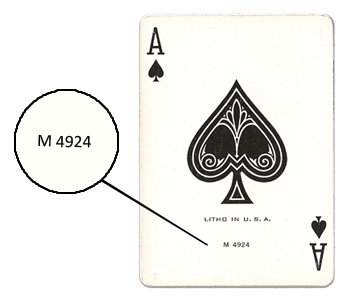This detailed close-up image features the Ace of Spades playing card. In the top left corner, there is a capital "A" followed by a spade symbol, while in the bottom right corner, the same "A" and spade symbol are inverted. A large, ornate spade dominates the center of the card, featuring intricate embroidery with a black and white outline and a smaller interior outline. Beneath this central spade, the text reads "L-I-T-H-B-N-U-D-S-D-A." Further below, in smaller letters and numbers, it says "M-4-9-2-4." The card's distinctive design and markings provide a rich visual detail.